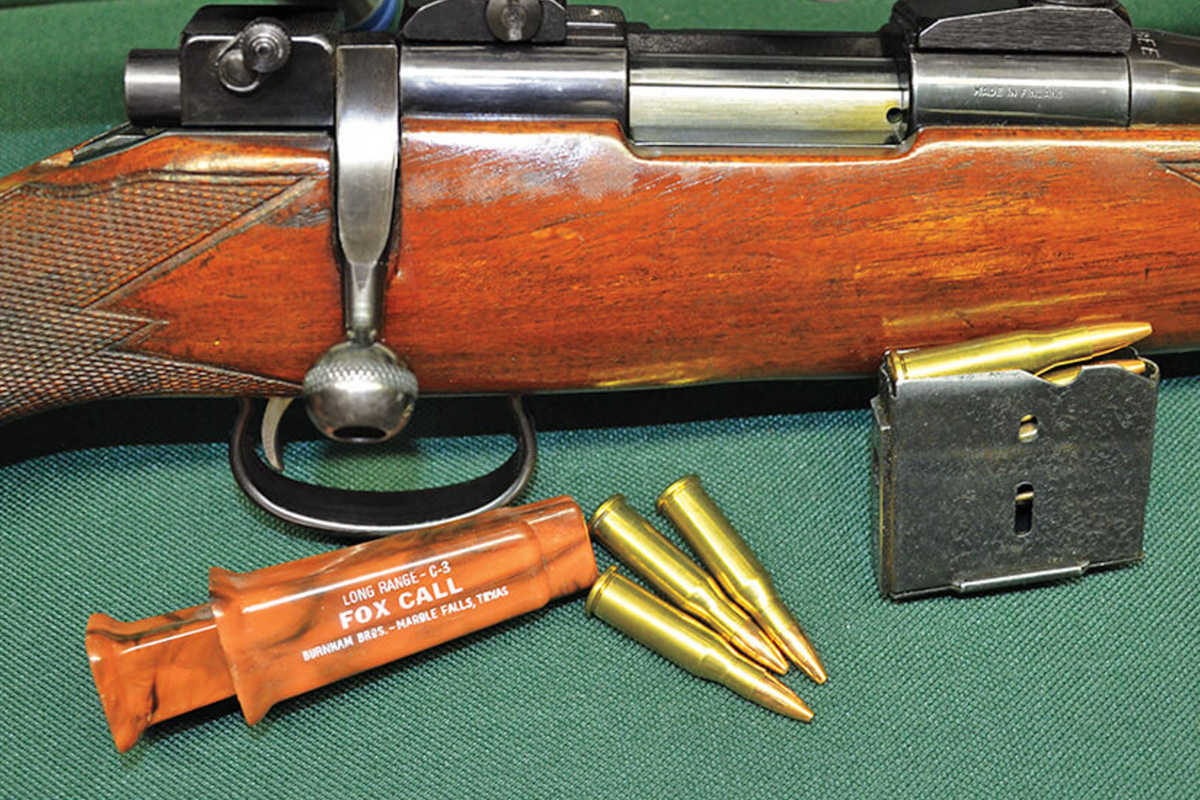The image depicts a well-worn rifle predominantly made of an old-style wood, marked with scrapes and areas where the finish has been worn off, indicating age and frequent use. The rifle is partially shown, focusing on the loading and trigger mechanism rather than the stock or barrel. The metal part where bullets are inserted is pewter-colored. Positioned on a green cloth beneath or in front of the rifle are a small orange packet labeled "Long Range C3 Fox Call" from Burnham Brothers Marble Falls, Texas, a bullet magazine capable of holding six bullets with three brass bullets laid out and one already loaded in the chamber. The arrangement highlights the brass bullets and the distinct components of the rifle, creating a scene of preparation or maintenance.